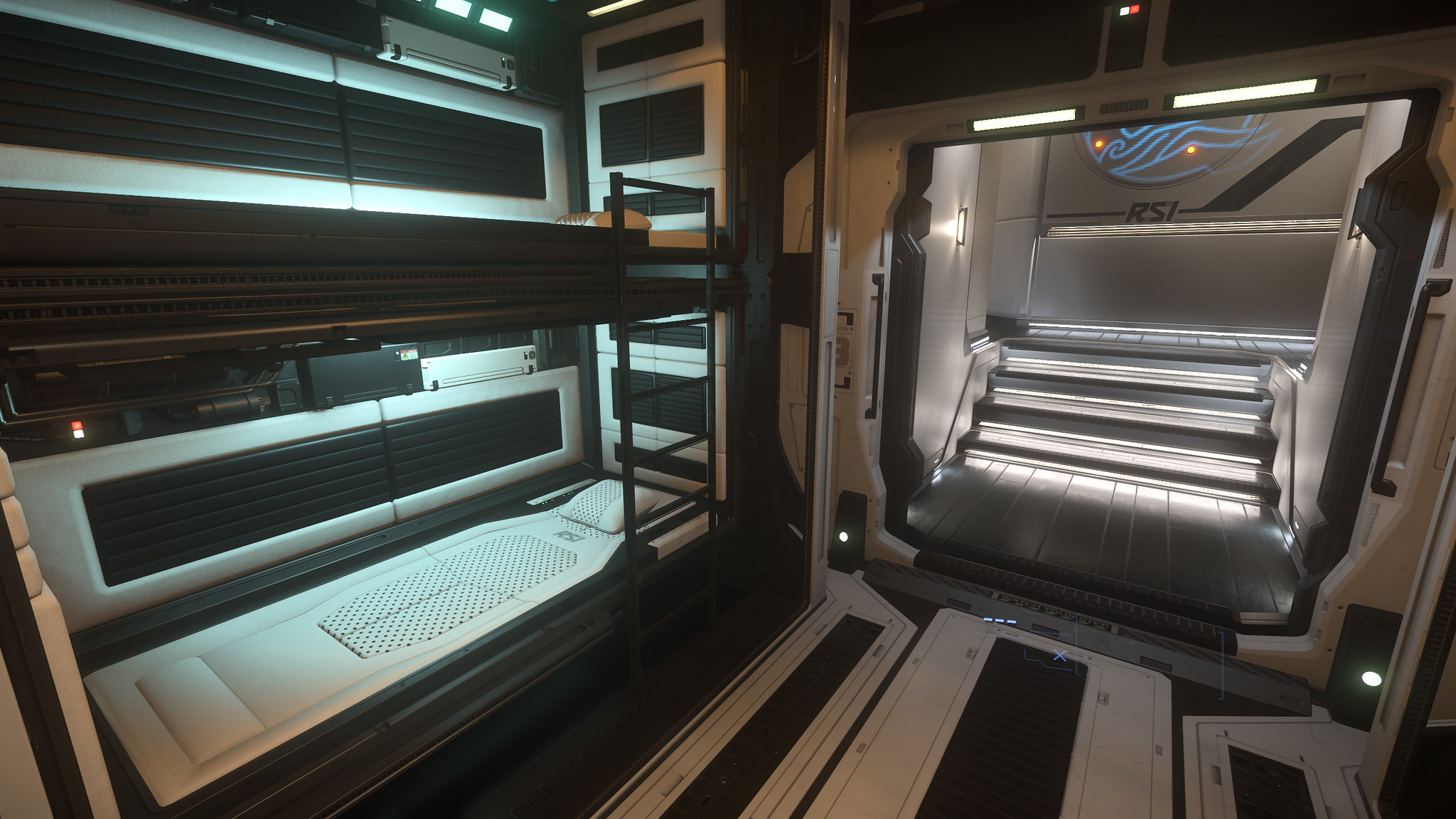This image appears to be a highly realistic, clean, and modern render, possibly from a video game or created using 3D software like Blender. The indoor scene, illuminated by artificial lighting, showcases a sophisticated, luxurious sleeping area with stacked sleeping pods reminiscent of a business hotel in Tokyo where space is at a premium. The pods resemble bunk beds without blankets, and their interiors boast white and black padded leather, integrated lighting, and satin metal frames, exuding a car-like luxury. There's also an integrated staircase and drawers, all contributing to the room’s sleek, futuristic aesthetic. A prominent stainless steel feature, possibly an air conditioning unit, and a neon sign with blue waves and the letters "RSI" add to the high-tech ambiance of the space.